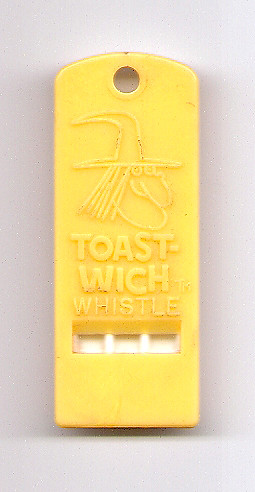The image showcases an antique toy whistle that appears to be from an old cereal box promotion. The whistle is small, rectangular, and made of yellow plastic with white details. The front of the whistle features an embossed image of a witch characterized by a traditional witch hat, stringy hair, a prominent nose, and a long chin. Below the witch's image, the text "Toast Witch Whistle" is clearly visible, likely indicating the name of the toy or its association with a cereal promotion. The image is tightly cropped, focusing on the detailed design of the whistle against a gray background. The top of the whistle includes a small hole, possibly for attaching it to a hook or string.